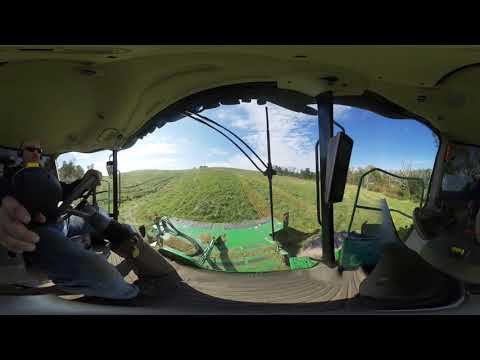The image captures the interior of a drivable piece of machinery, presumably a tractor or another type of farm equipment, since it is surrounded by a green field. The interior is predominantly dark, with a black dashboard and a white canopy overhead. To the left, there is a bald driver wearing dark-colored sunglasses and yellow neckwear, likely part of his shirt. His left hand is on the steering wheel, while his right hand is on a gear shift. Visible through an open window is a vast, green, grassy field extending towards a large hill covered in the same lush greenery. The vibrant blue sky above is dotted with white, fluffy clouds. A dark post and a railing are seen on the right side of the image, framing the scene from within the vehicle.